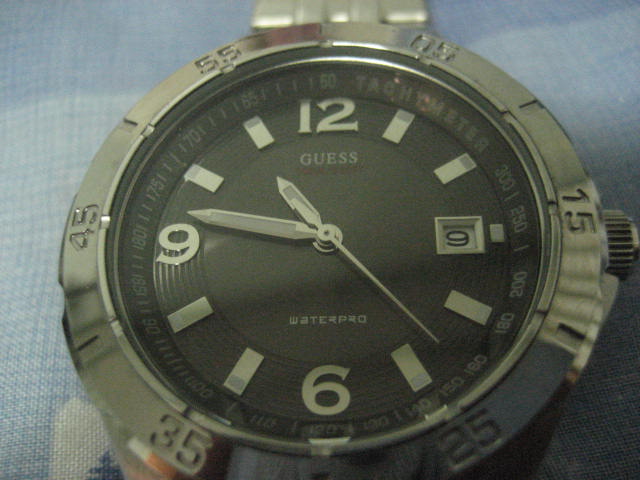The image showcases a detailed close-up of an elegant wristwatch. The background features a blue and white checkered surface with intersecting vertical lines and rows, creating a visually appealing contrast to the watch. The wristwatch itself is distinguished by a large circular face, encased by a metallic bezel adorned with numerical markers. The face of the watch is protected by a clear glass cover, revealing the numerals 12, 6, and 9—although, unusually, the numeral 9 appears twice, instead of where the 3 should be. Smaller numbers are meticulously inscribed in black just inside the outer silver bezel, adding another layer of intricacy to the design. Silver hands gracefully indicate the time, adding a touch of sophistication to the timepiece.